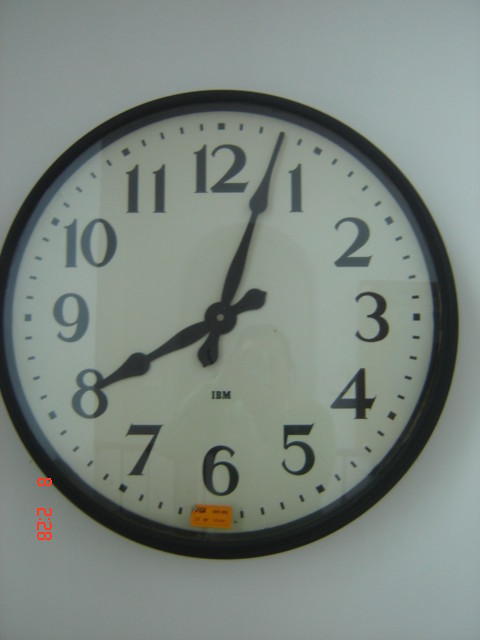This image features a simplistic, round clock set against a white wall. The clock's design includes a black frame with a white face, black numbers ranging from 1 to 12, and black hour and minute hands, but no second hand. The clock's time reads 8:03. At the bottom, near the number 6, there's an orange sticker that might indicate it's for sale, as well as the letters "IBM" in black text. Additionally, red numbers "8228" are visible in the bottom left corner of the image, possibly from a timestamp or marking. The clock occupies about 70 percent of the image and has a glass cover that reflects a person holding a camera, who appears to be wearing a green shirt and has a beard.